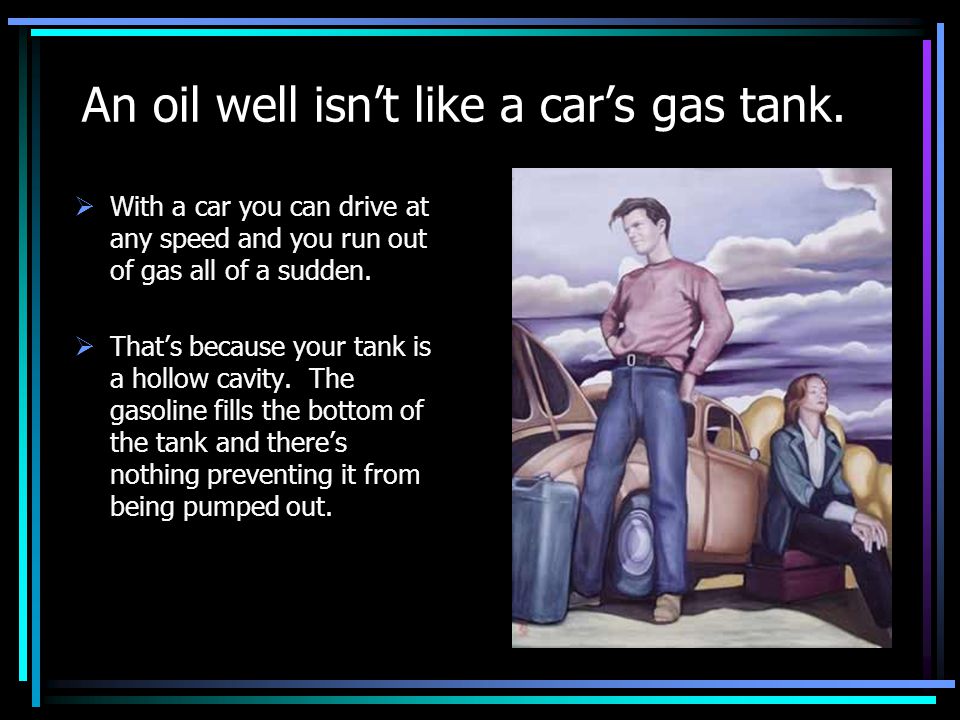This image, resembling a PowerPoint slide with an educational theme, features a black background bordered by thin lines with a gradient of blue, green, and purple. The top of the slide displays large white text stating, "An oil well isn't like a car's gas tank." Beneath this, two bullet points clarify the concept with white text: "With a car, you can drive at any speed and you run out of gas all of a sudden," and "That's because your tank is a hollow cavity. The gasoline fills the bottom of the tank and there's nothing preventing it from being pumped out." On the right side of the slide, there is a cartoony illustration of a man and a woman who appear to have run out of gas, standing by their broken-down car on the roadside. The man, looking unhappy, is dressed in a red shirt and blue pants, while the woman, who has her eyes closed, is sitting on a suitcase. The scene includes a simplistic background suggesting an outdoor setting.